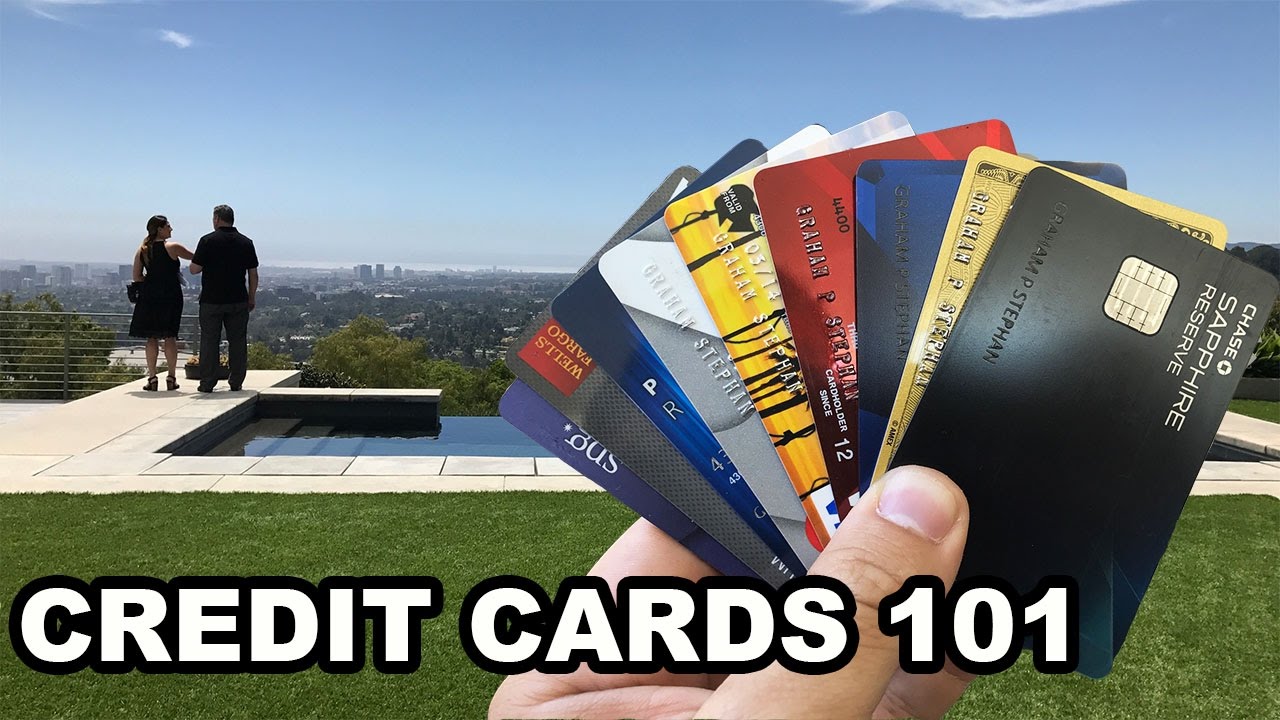The image appears to be a marketing visual for a blog or podcast titled "Credit Cards 101," prominently displayed in large white sans-serif text with a thick black outline at the bottom left corner. Dominating the foreground is a left hand fanned out displaying eight diverse credit cards, including identifiable ones such as the Chase Sapphire Reserve and Wells Fargo cards. The background transitions from a vibrant green lawn to a sleek infinity pool set against a cityscape that resembles Los Angeles. To the left of the pool, a man and a woman dressed in black attire—she in a sleeveless dress with chunky high heels and he in a black polo shirt with charcoal gray slacks—stand gazing at the distant skyscrapers under a clear blue sky adorned with slight wisps of clouds.